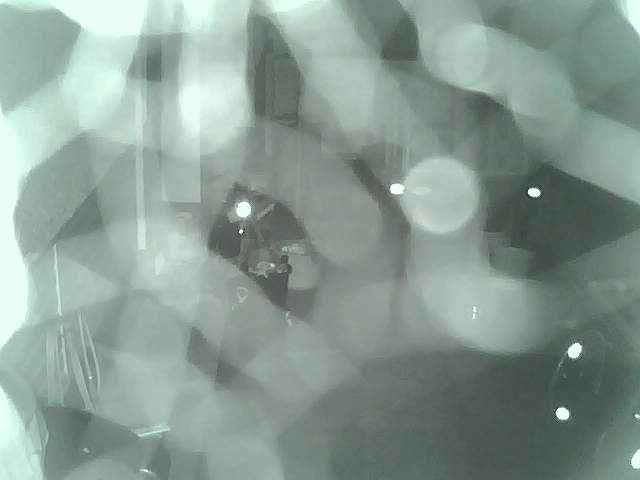In this extremely blurry and indistinct image, we observe a rectangular shape that is slightly wider than it is tall, giving it an approximate width-to-height ratio of 60:40. The image is predominantly tinted green, featuring thick, wavy lines reminiscent of squiggles or possibly worms, spread chaotically across the frame. These lines vary in opacity, creating patches of a soft mint green where they overlap more densely. Amidst this chaos, there are sporadic patches of white light interspersed throughout the image, hinting at some form of illumination. In the background, though details are obscure, one can vaguely discern what appears to be a camera positioned on a black desk. Additionally, the image might include elements suggestive of a room's interior, featuring what could be white barrels and possibly a white bucket.